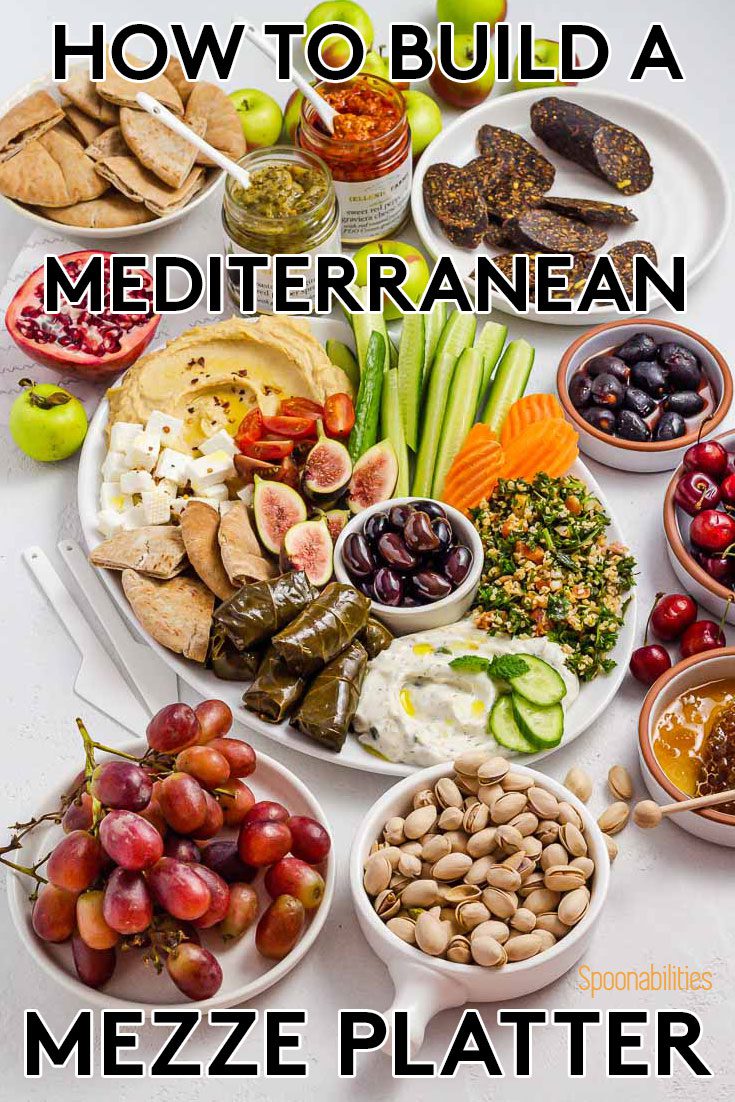The vertical rectangular image features an appetizing display of assorted Mediterranean foods arranged in different white dishes on a gray background. Dominating the top of the image, in bold black letters, is the text "How to Build a Mediterranean Mezze Platter." Central to the composition is a large oval white platter filled with an array of vibrant vegetables including sliced cucumbers, carrots, celery, and what appears to be garbanzo beans, possibly hummus, and diced mozzarella cheese. Surrounding this central platter are additional white bowls and plates, each containing a variety of items. In the foreground to the left, there's a prominent bowl of red grapes and beside it, a white bowl of pistachios. Also present are a bowl of cherries, a cut pomegranate, and black olives. Additional dishes include a plate with some kind of sausage, two jars of sauce, and scattered pieces of green apples. The abundant assortment of fresh ingredients creates an enticing and visually appealing presentation.